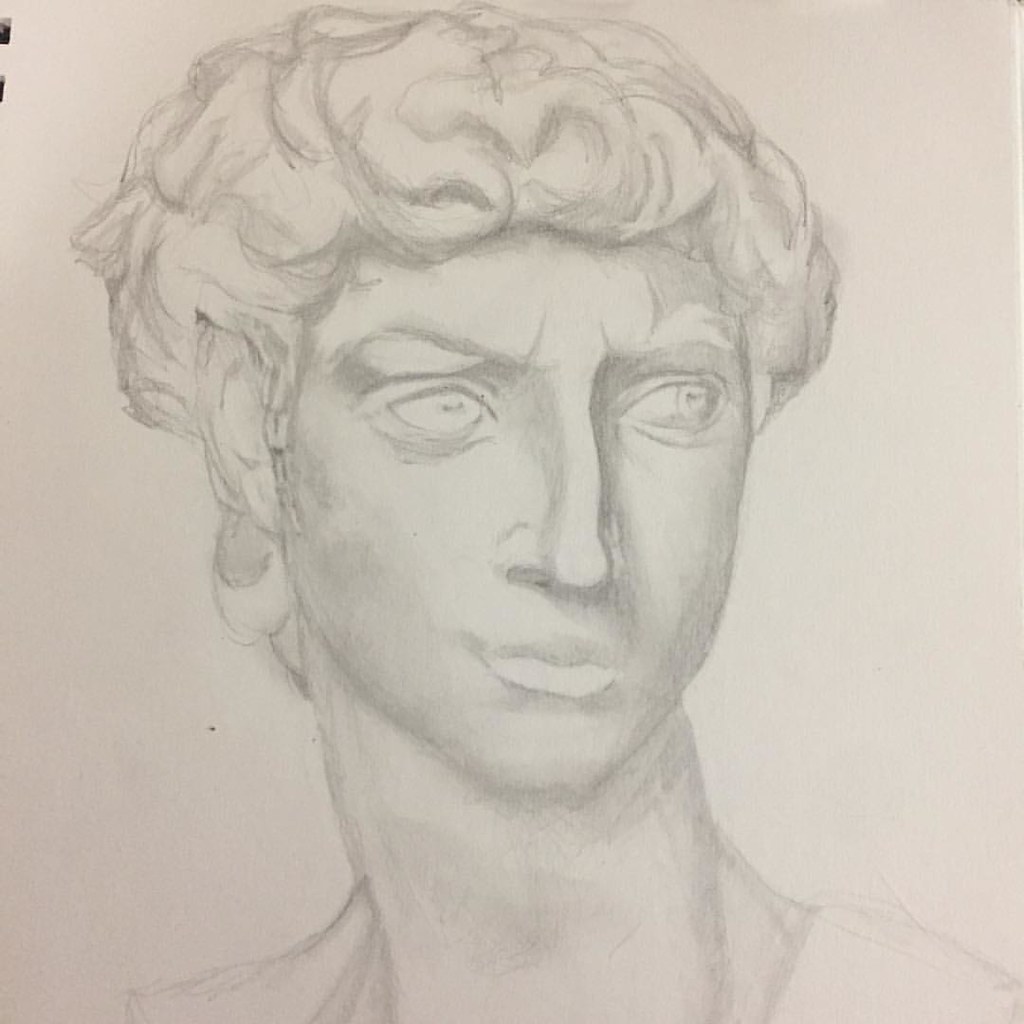This image features a meticulously detailed drawing of an individual whose gender is ambiguous. The person depicted has a thick, curly, and wavy mane of hair, which is cut to fall just over the ears while extending a bit longer down the back. The subject is portrayed in profile, their gaze fixed intently on an unseen object, imparting a pensive, contemplative expression. This expression is accentuated by subtle lines on the forehead, suggestive of a furrowed brow indicative of deep thought or puzzlement.

The person's nose is distinctively bony with a noticeable bump in the middle, adding character to the face. The lips are relatively full, contributing to the overall well-proportioned and shapely appearance of the face. The artist has skillfully utilized pencil shading to enhance the contours and features, creating a realistic and textured effect.

The neck of the individual is elongated, further emphasizing the thoughtful demeanor. The ambiguity of clothing is maintained as the shading leaves it unclear whether the person is dressed or not. The entire drawing is set against a beige background, adding warmth to the image and providing a gentle contrast to the pencil work. In the upper left-hand corner, two small black areas are visible, adding an intriguing and mysterious element to the composition.